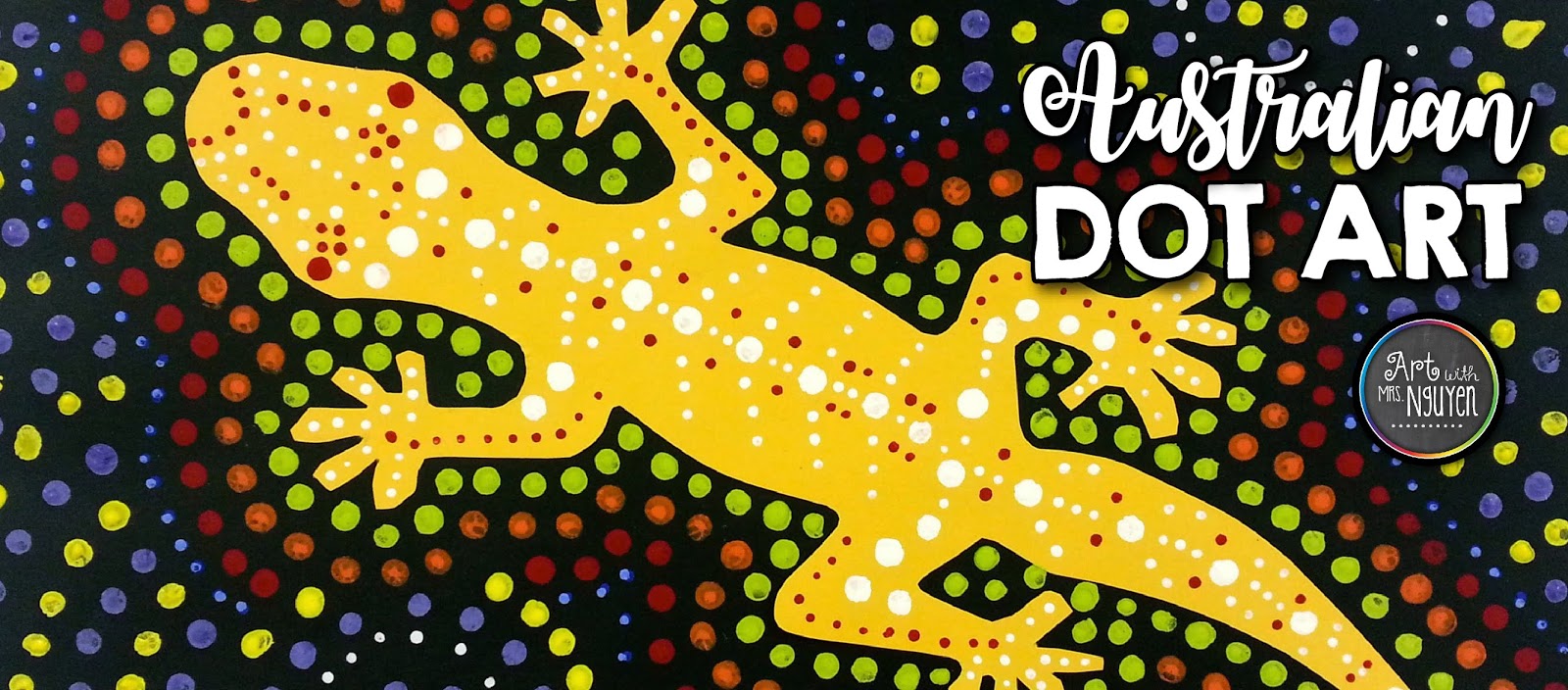The image is an artistic representation titled "Australian Dot Art," with the text prominently displayed in white— "Australian" in a cursive script and "dot art" in all caps. Beneath this text, on the upper left corner, there is a circular logo stating "Art with Mrs. Wynne" (or "Miss Nguyen") in curly font. The main subject of the artwork is a lizard or gecko, depicted with a yellow outline. Inside the lizard, there are red and white dots that accentuate its body. The lizard itself is set against a very dark blue background, with all four feet visible, each adorned with five toes. Encircling the lizard are successive rings of colored dots, starting with yellow dots closest to the lizard, followed by rows of orange, red, tinier blue, and intermingled yellow and purple dots. The overall composition creates a vibrant and detailed mosaic-like effect.